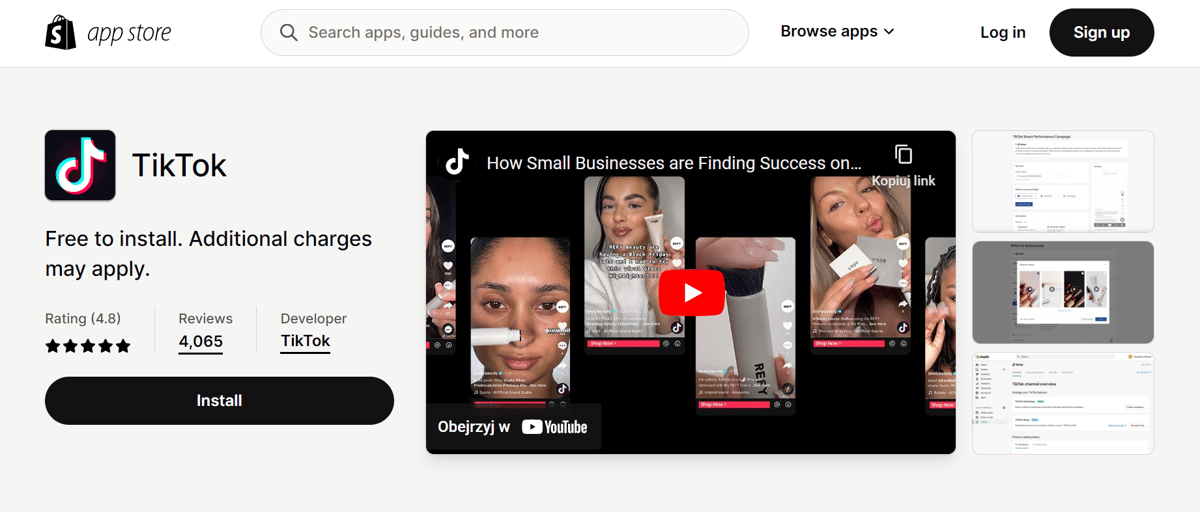A cropped screenshot of the App Store app interface is displayed. At the top of the page, there is a centered search bar with the placeholder text "Search Apps, Guides, and More." To the right of the search bar is a black drop-down menu labeled "Browse Apps." Further right are the options to "Log In" and "Sign Up." The background of the page is gray.

On the left side of the screen is a TikTok icon, with the text "TikTok" immediately to the right. Below this, it reads "Free to Install, Additional Charges May Apply." In the bottom left corner, the app's rating is shown as 4.8 stars out of 5 based on 4,065 reviews. Next to this, it specifies that the developer is TikTok, displayed in black text. An "Install" button in black is positioned below this information.

Centrally located on the page is a YouTube video titled "How Small Businesses are Finding Success on TikTok," featuring a thumbnail image. The bottom left corner of the video shows the username of the creator along with the YouTube logo.